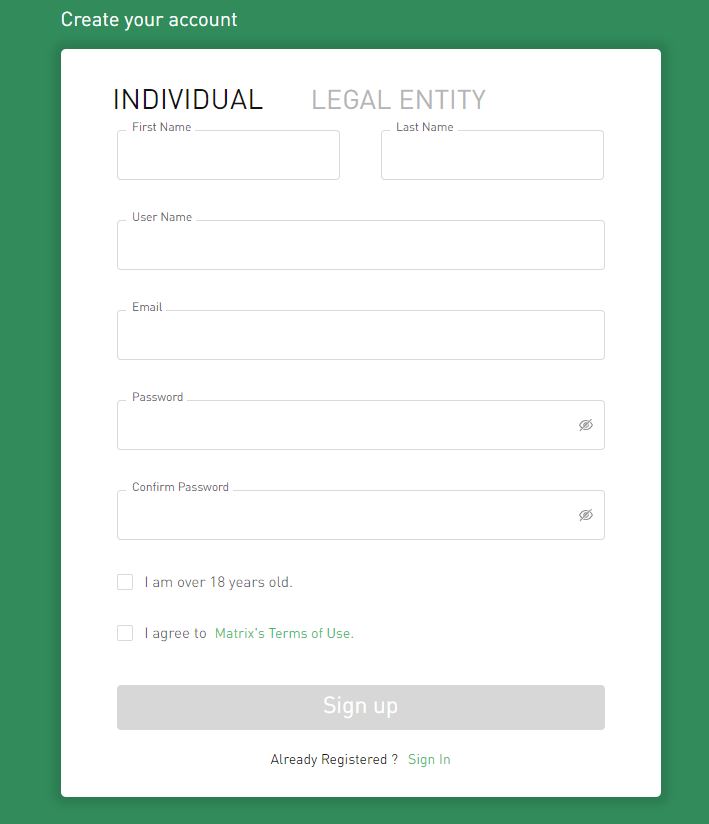A screenshot of a web page displaying a "Create Your Account" form for a website named Matrix. The entire background of the web page is green. In the center of the page, there is a white input box designed for user information. The form provides options to sign up as an individual or a legal entity, though the latter option is currently grayed out. Within the white box, there are fields to enter a first name, last name, username, email, and password. Both password fields include eye icons with slashes, indicating users can toggle visibility. Below the input fields, there are two checkboxes: one confirming the user is over 18 years old, and another agreeing to Matrix's terms of use. A green "Next" button is present, alongside a grayed-out "Sign Up" button with white text. At the bottom of the form, there is a prompt reading "Already registered?" in black and white, followed by a green-text "Sign In" link. The entire scene bears a striking thematic resemblance to the aesthetics of the "Matrix" movie from years ago, though it is a standard sign-up page for Matrix's website.